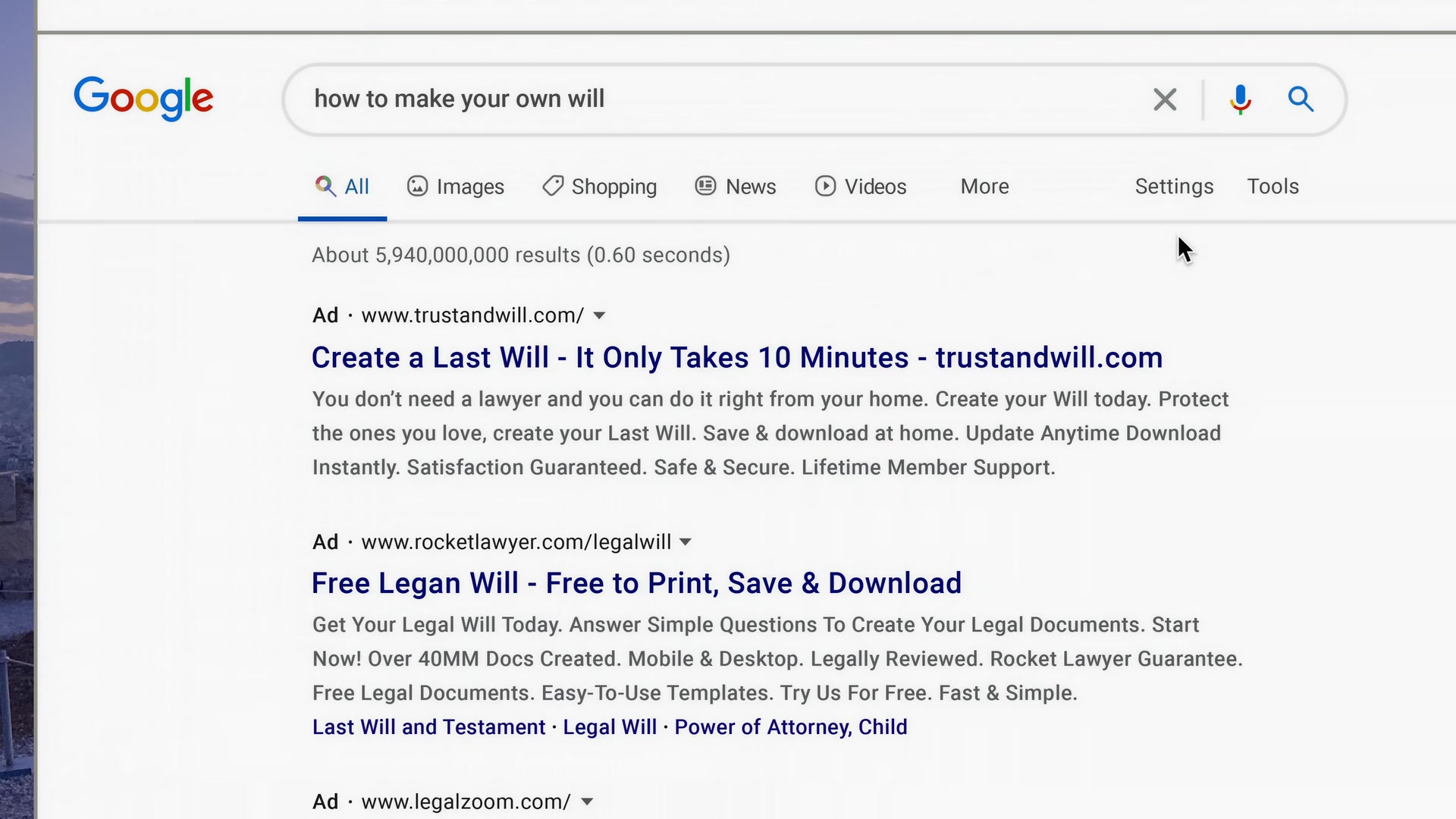A screenshot of a Google search results page shows a light gray background with a vertical, gradient bar on the left side displaying various shades of purple and a hint of black. At the top of the screen, a black line features the Google logo in its signature multicolored lettering, followed by the search query "how to make your own will" within a search bar. Adjacent to the search bar are icons of an 'X', a microphone, and a magnifying glass.

Below the search bar, another magnifying glass icon precedes the word "All," which is underlined in blue. Directly beneath this blue line is a continuous gray line stretching across the screen. Further down, the options "Images," "Shopping," "News," "Videos," "More," "Settings," and "Tools" are listed in sequence.

An advertisement follows, containing small text that includes "Ad" alongside a website link: "create a last will – it only takes ten minutes – trustandwill.com." The ad includes additional, smaller text that is difficult to read. Another section labeled "Ad" mentions "Free legal will – Free to print, save and download," accompanied by a brief paragraph in black text and a few blue words. At the very bottom of the image, the word "Ad" and the website are repeated.